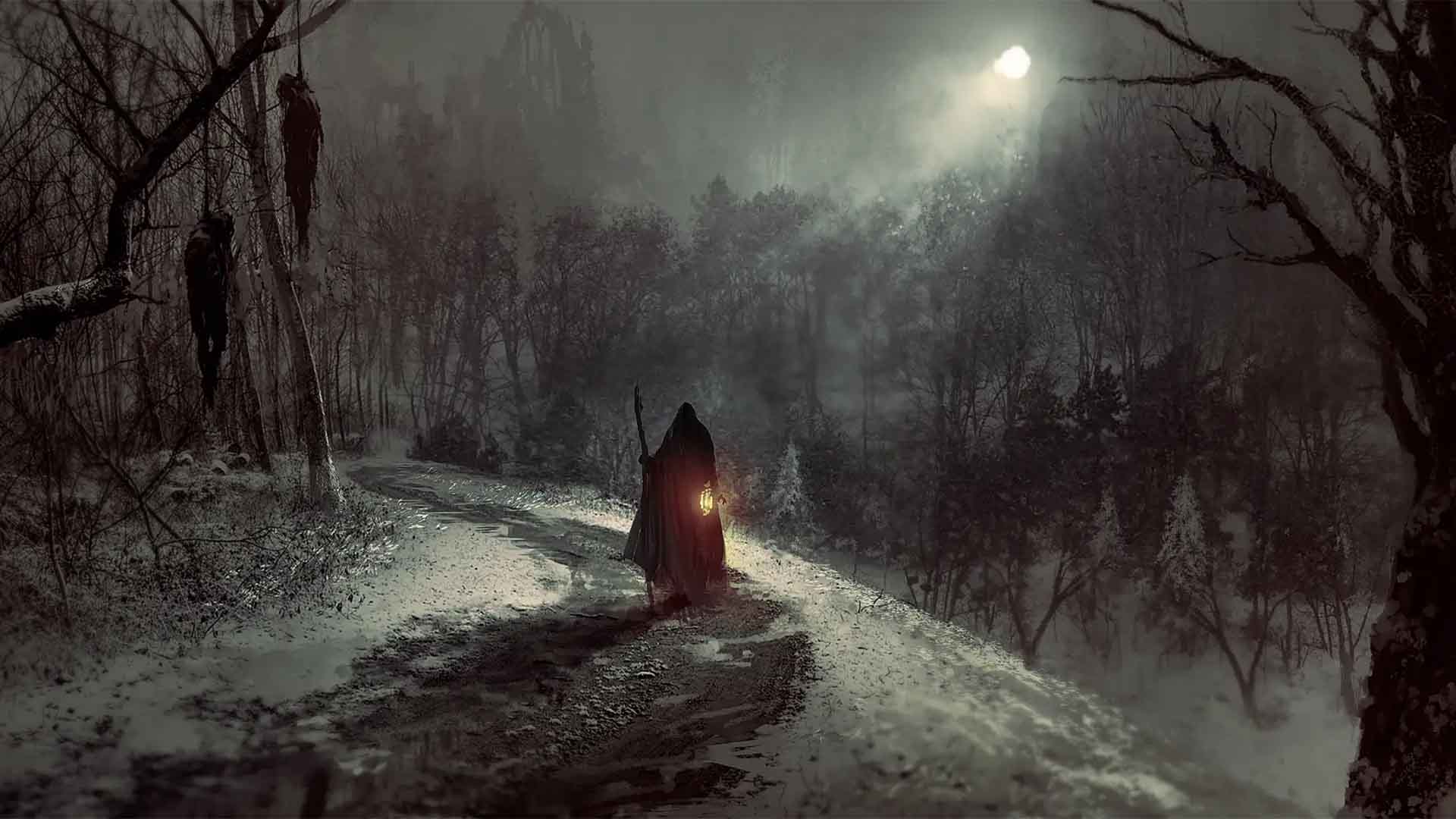The image is a rectangular painting, approximately six inches wide and three inches tall, predominantly in grayscale. It depicts a nighttime scene illuminated by a bright, reflective moon in the upper right-hand corner, casting an ethereal glow over the landscape. At the center of the painting, a dirt walking path, originating from the lower left corner, winds up a hillside before switching directions twice. Along this eerie path, a cloaked figure garbed in black walks, carrying a staff in one hand and a lantern in the other, their light cutting through the darkness.

To the left of the cloaked figure, barren and leafless trees stand ominously against the night sky. Among these trees hang two deceased bodies, draped in rags and suspended by ropes around their necks, with no visible blood, adding to the macabre atmosphere. On the right side of the path, the hillside slopes away, revealing the large trunk of another barren tree. Further in the background, more leafless trees stretch towards a decaying castle ruin in the upper left corner, enhancing the eerie and abandoned feel of the scene. A faint fog rises through the valley below, shrouded in moonlight, completing the haunting depiction.